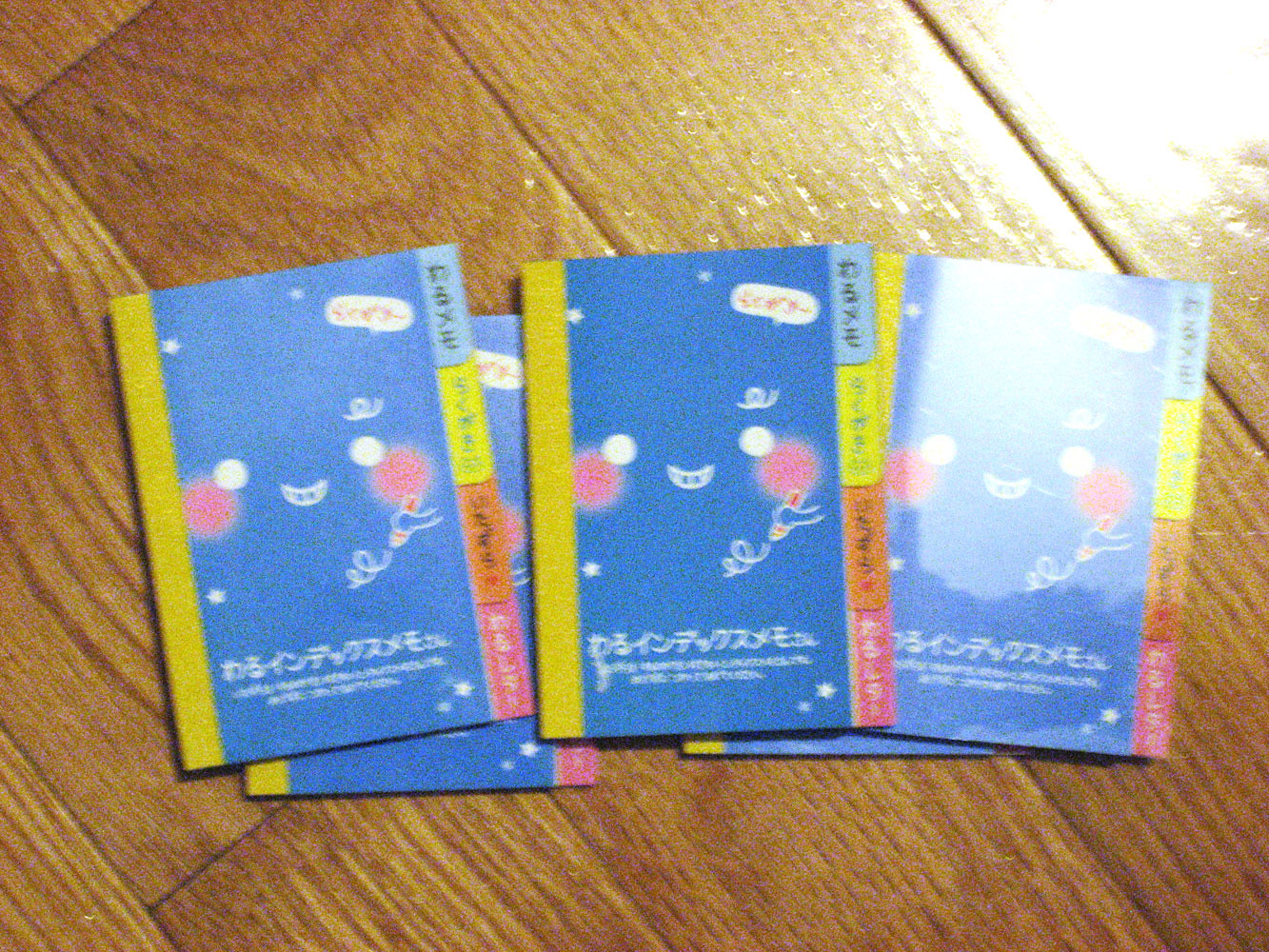This photo captures five small booklets placed on a wooden slat floor, slightly out of focus due to a bright white light emanating from the top left corner, which partially obscures the leftmost booklet. All five booklets are identical and predominantly blue, featuring a prominent yellow strip on one side and a series of colorful tabs—brown on the left, green, yellow, and red on the right. The center of each booklet's cover showcases an illustration resembling a smiley face with two white eyes, a mouth, and two red cheek-like spots. Accompanying this friendly design is text in Japanese, visible at both the bottom and within the multicolored tabs, suggesting they contain Japanese writing or characters. The booklets are quite small, likely half the size of a standard A4 sheet, and their purpose remains unclear to non-Japanese speakers.